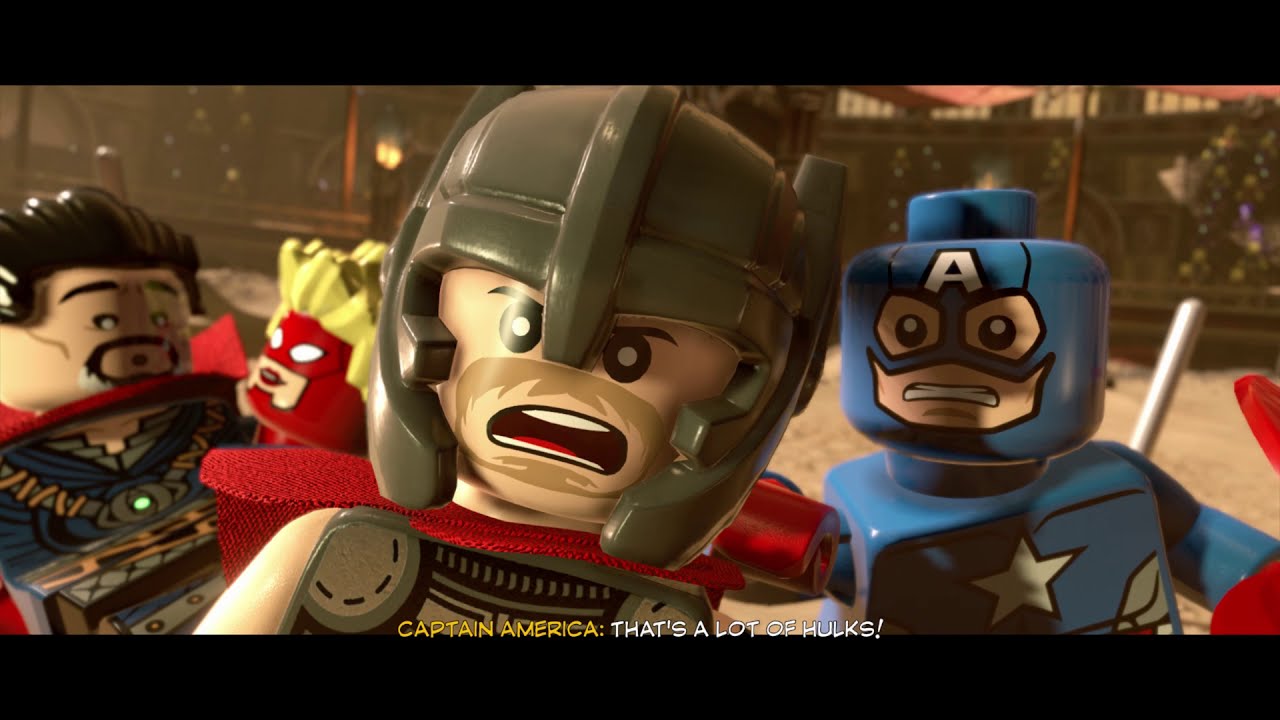The image appears to be a screenshot from a Lego-themed Avengers movie or video game, framed with a black border at the top and bottom. Four Lego characters are prominently featured. The central focus is a Lego character resembling Thor. He stands out with his brown helmet, light brown goatee, grey body armor, and red cape, visible from the shoulders up. Just to Thor's right is a Lego version of Captain America, clad in his iconic blue suit with a white star on his chest. On the far left is a character identified as Doctor Strange, distinguished by his black spiky hair, white goatee, red cape, and black facial hair. To his right, closer to Thor, is another character with blonde spiky hair and a red mask, likely Miss Marvel, as her mouth is exposed and her yellow hair peeks through. The scene includes a caption at the bottom that reads, "Captain America, that's a lot of hulks!" suggesting dialogue from the movie or game.